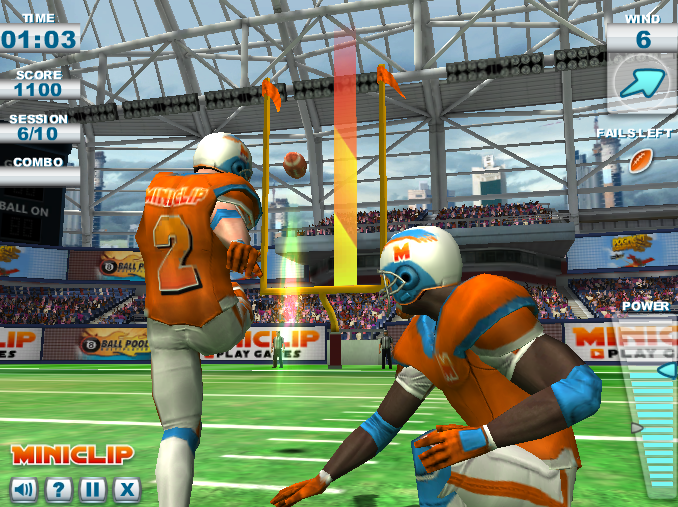This screenshot, taken from a classic video game, showcases the charmingly rudimentary 3D graphics characteristic of early gaming technology. Exhibiting low-polygon models with pixelated edges, the visuals capture the essence of the era’s simplified design. The scene depicts a football game in which a player from a team dressed in vibrant orange jerseys and white pants with an orange stripe kicks a field goal. The football is frozen midair, having just been launched by the kicker. His leg remains elevated from the kick, emphasizing the motion. The yellow, U-shaped goal post stands prominently in front of the players, providing a stark contrast to the blurred, simplistic background.